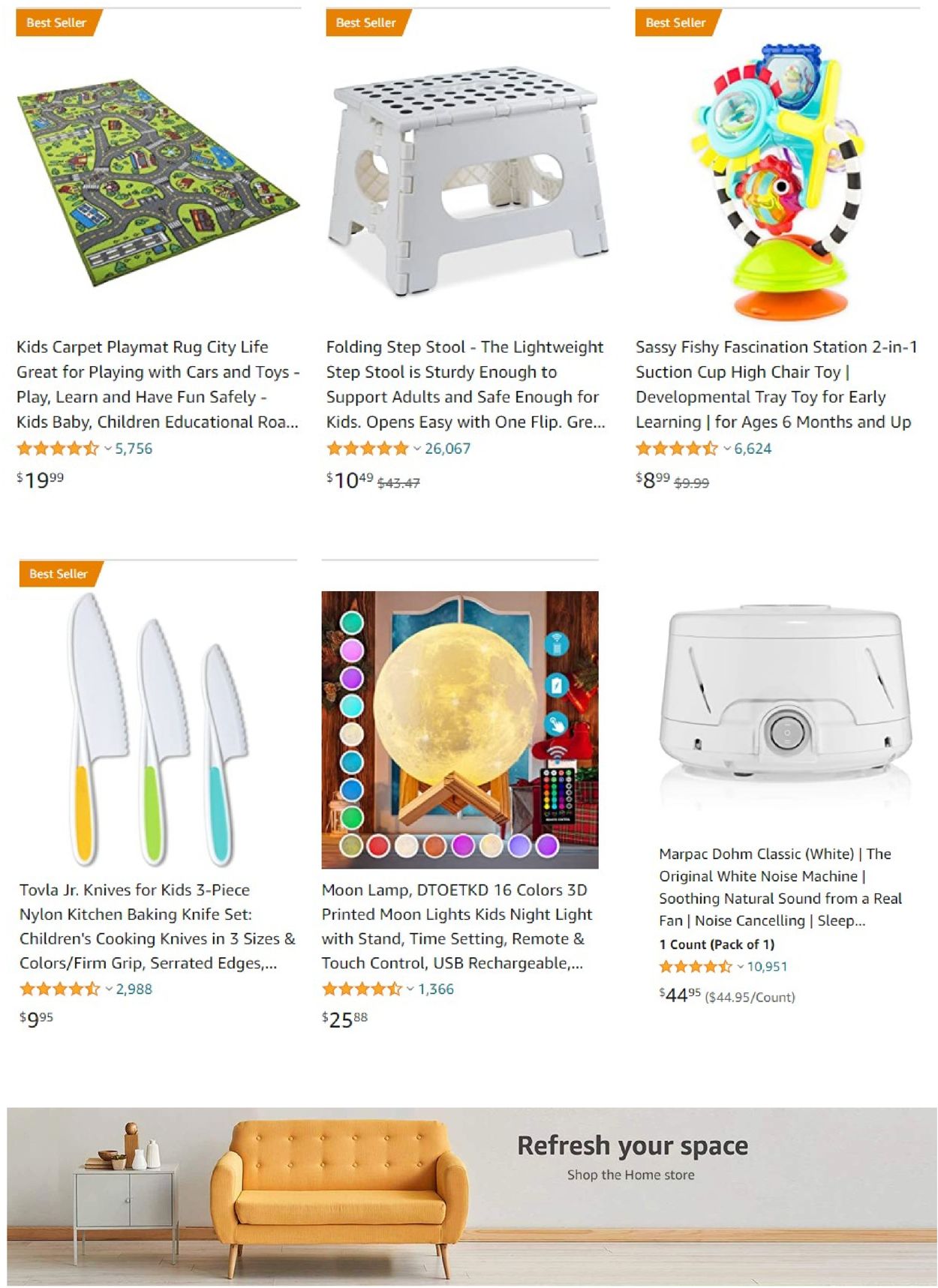This screenshot from a shopping website features a grid of six items, arranged in a 3x2 formation. Notably, four of these items are marked as best sellers. 

In the first row, from left to right, we see:
1. A Kid's Carpet Playmat Rug designed for play activities.
2. A Folding Step Stool, ideal for reaching higher places.
3. A Sassy Fishy Fascination Station, a 2-in-1 suction cup high chair toy meant to entertain infants.

In the second row, the first item is the final best seller:
4. Tovala Jr. Knives for Kids – a three-piece nylon kitchen baking knife set specifically designed for children's cooking, featuring three different sizes, firm grip handles, and serrated edges, priced at $9.95.

The remaining two items on the second row are:
5. A Moon Lamp with 16 colors, which is a 3D-printed kids' nightlight equipped with time settings, remote control, and touch control features.
6. A White Noise Machine, branded as the Classic White Original, designed to provide soothing sound for better sleep and relaxation.

This well-organized grid offers a variety of child-friendly and practical household items.